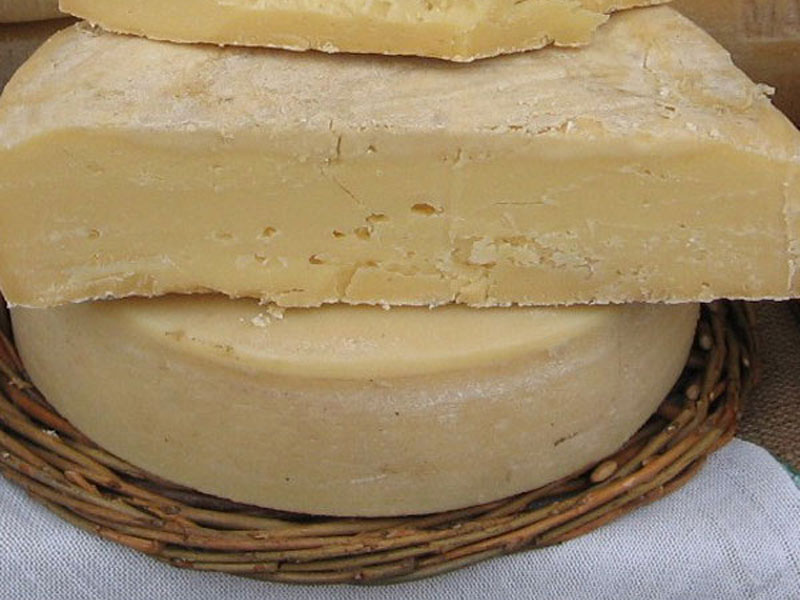The image features a close-up shot of three blocks of cheese arranged on a brown woven wicker plate, which rests on a piece of white linen. The bottom block of cheese is cylindrical and creamy yellow with a whitish, dusty exterior. The middle block is square and slightly crumbly, resembling parmesan, while the third block, only partially visible, appears to be cut off at the top of the frame. The cheeses display some holes and streaks, indicative of their texture. The wicker plate, which resembles a round, woven wooden basket, sits atop a white tablecloth, partially visible beneath it. The background of the image has a warm brown tone, complementing the rustic presentation of the cheeses.